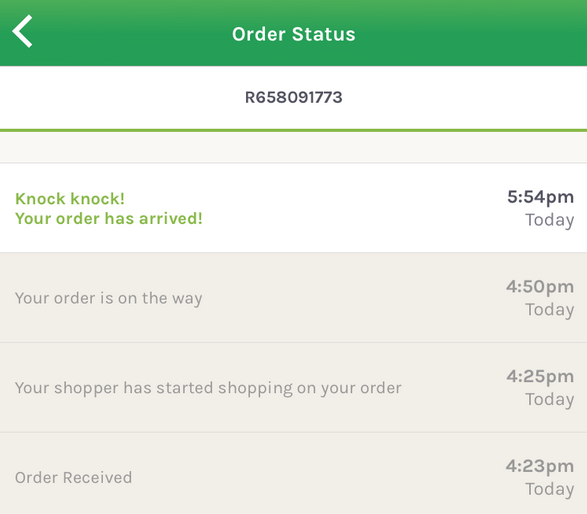The image depicts a digital order status notification, typically seen on a tablet or computer. At the top of the notification is a green box with white text reading "Order Status." In the top left-hand corner, an arrow points left. Below the "Order Status" heading is an order number displayed in black text on a white background: "R658091773."

Beneath the order number, a green line separates the header from the rest of the notification. Below this line is a gray box containing the message "Knock Knock! Your order has arrived!" written in green text aligned to the left. The notification also specifies the delivery time as "5:54 p.m. today," with "5:54 p.m." in black text and "today" in gray.

Further down, three status updates in gray text are listed:
1. "Your order is on the way, 4:50 p.m. today."
2. "Your shopper has started shopping on your order, 4:25 p.m. today."
3. "Order received, 4:23 p.m."

This detailed tracking information is indicative of a grocery delivery service, such as Instacart, providing real-time updates on the progress and completion of a customer's order.